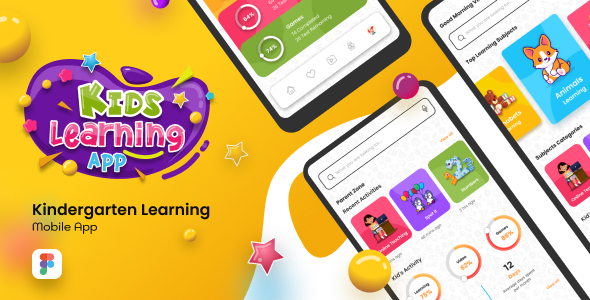This image is an advertisement for a kindergarten learning mobile app set against a yellow background. On the left side, a 3D purple bean-shaped graphic prominently features the words "Kids Learning App," adorned with small stars and yellow balls. 

In the center at the top, the bottom portion of a cell phone is visible, displaying horizontal yellow, pink, and green stripes. Directly beneath this, another cell phone is positioned at an angle, showcasing an empty search bar at the top, followed by the label "Parent Zone." This section includes three graphic illustrations in pink, purple, and green.

On top of this angled cell phone lies a large yellow circle labeled "Kids Activities," with round circles inside displaying various percentages. Finally, in the top right corner, a third cell phone, aligned sideways, greets with "Good Morning" and lists "Top Learning Subjects," accompanied by different selectable boxes.

The overall design is vibrant and interactive, blending educational themes with visually engaging elements to appeal to both children and parents.